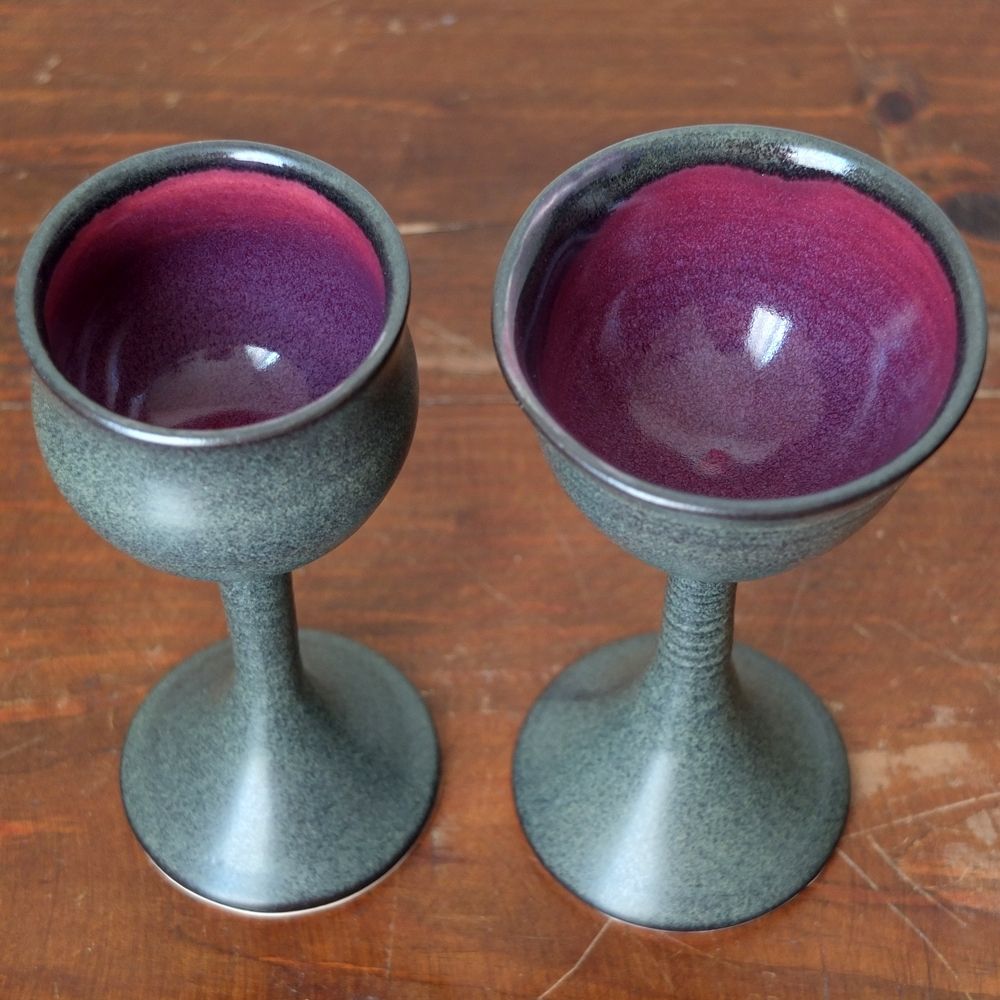This color photograph captures two handmade clay goblets from an overhead angle, revealing their maroon-purple interior glazes. Both goblets rest on a dark hardwood table, which shows slight etching, contributing to the rustic atmosphere. The exteriors of the goblets showcase a glossy, slate-gray finish, contrasting with the vibrant inner hues. Although both goblets share a similar aesthetic, they differ slightly in shape, with the right goblet featuring a marginally wider cup. The kiln-fired craftsmanship is evident in their unique forms and the careful application of the glaze.